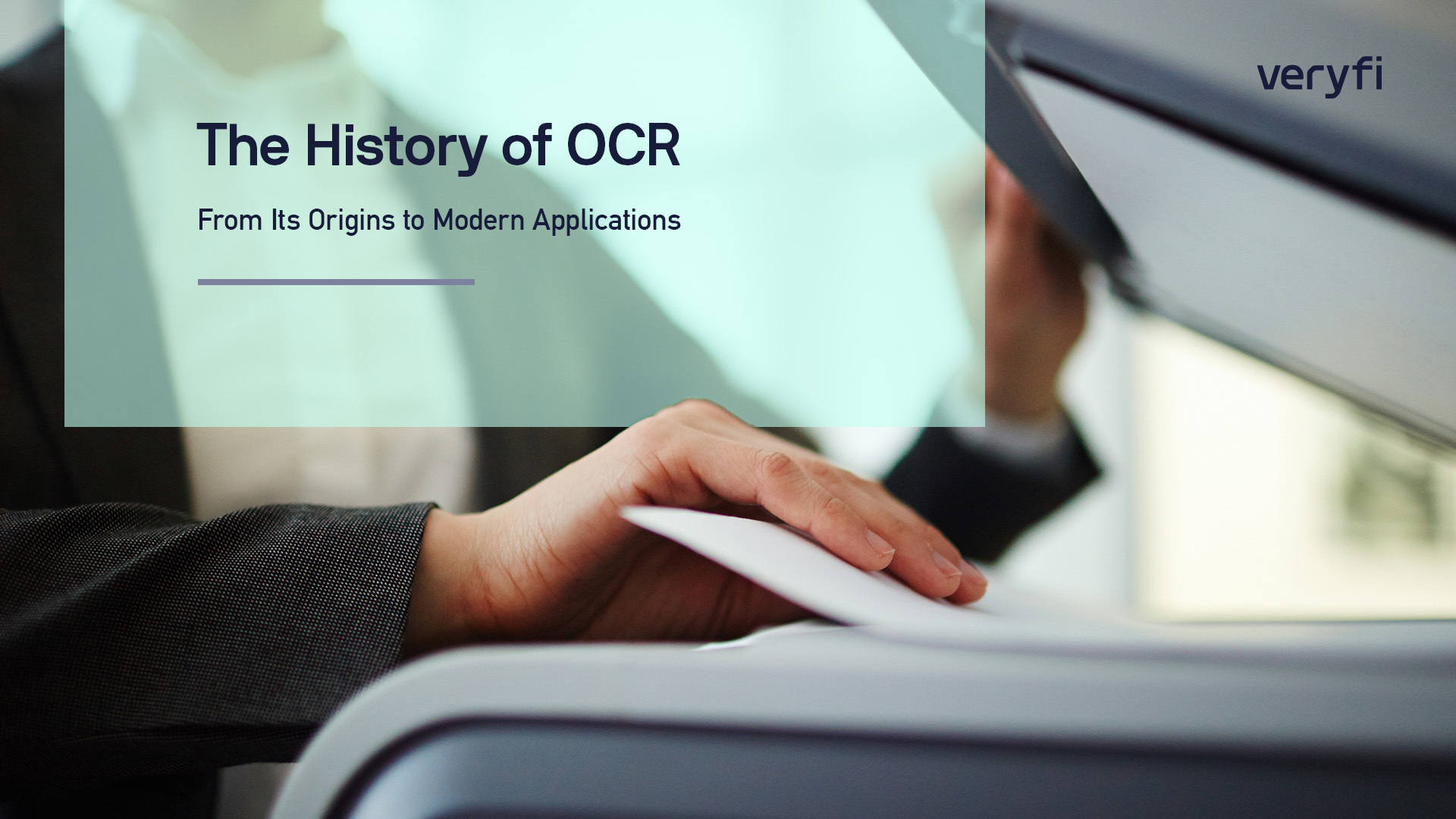In this image, a person dressed in a dark gray suit jacket and a white button-down shirt is seen inserting a piece of paper into the scanner bed of a gray and white copy machine. The lid of the copier is open, revealing a white panel underneath. The individual's hands are clean and appear to be in the process of either placing or folding the paper onto the scanner. In the upper right-hand corner of the image, the text "Verify" spelled out as V-E-R-Y-F-I is prominently displayed in blue. Meanwhile, in the upper left-hand corner, there is an opaque teal text box that reads, "The History of OCR, From Its Origin to Modern Applications." This box slightly overlaps with the hand, partially obscuring the background. The overall setting hints at a professional environment, possibly an office, suggested by the out-of-focus lighting in the background.